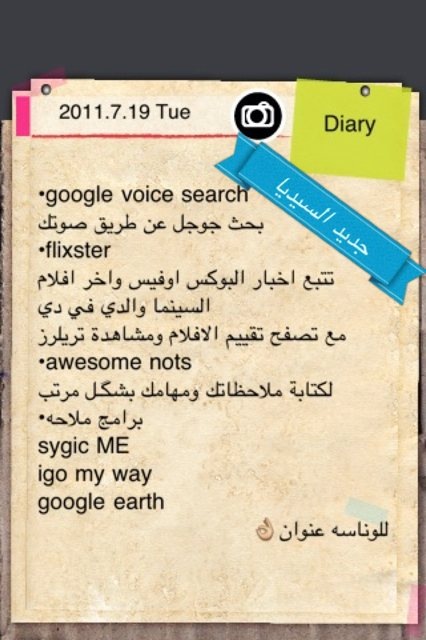The image is a digital representation of a document-themed user interface with a timestamp in the upper left corner that reads "2011.7.19 Tuesday," underlined in red. The layout is in portrait mode, set against a dark gray background that fades into a lighter, creamy marble towards the bottom, where a strip of pink scotch tape appears in the bottom right-hand corner. A black circle icon resembling a camera is placed near the date. Adjacent to this, in the upper right corner, is a green post-it note labeled "diary" in black text. The middle of the document features a blue ribbon extending from the center towards the right, displaying some Arabic text. Below this ribbon, a list of items is presented: Google Voice Search, Flixster, Awesome Knots, SYGIC, I-GO My Way, and Google Earth, interspersed with additional Arabic text.